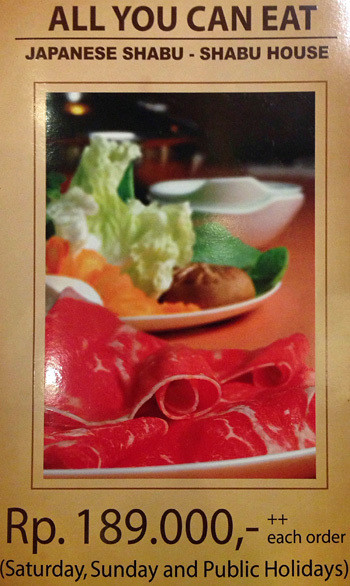This advertisement features a vertically aligned rectangular image with a medium brown background. At the top, in all caps black letters, the slogan "ALL YOU CAN EAT" is prominently underlined. Below this, it reads "Japanese Shabu-Shabu House." The centerpiece of the advertisement is a large vertical rectangular photo showcasing a tempting array of food. At the bottom of the photo, rolled red and white meat, possibly prosciutto or beef carpaccio, is displayed. A central plate holds what appears to be lettuce, along with indistinguishable brown and orange items that may be vegetables such as carrots or other garnishes. In the backdrop, a white bowl or dish is visible, adding depth to the scene. The price, "RP 189.000" is specified near the bottom, accompanied by two plus signs indicating additional charges per order. This is followed by the text in parentheses, "Saturday, Sunday, and public holidays," written in either black or dark brown font. This detailed and inviting sign serves as a promotional menu insert for the restaurant's buffet offerings.